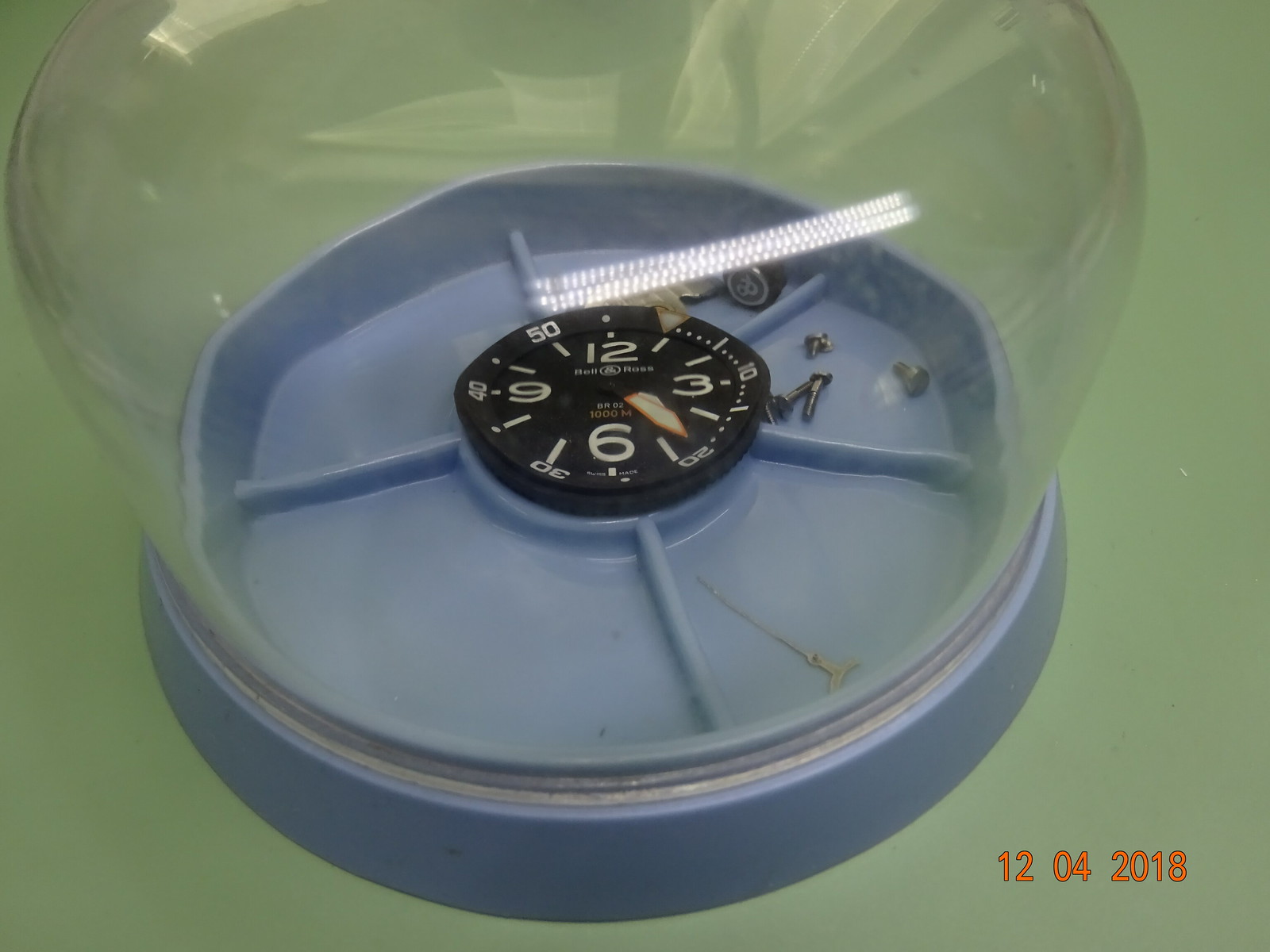A rectangular photograph in landscape orientation features a mint green background. In the bottom right corner, the date "12-04-2018" is displayed in orange text. Central to the image is a blue plastic circular object with roughly one-inch-high sides, resting on a flat black circular base. Atop this structure is a bulbous, transparent globe, resembling the shape of a light bulb, though it is unclear whether it is made of plastic or glass. Within the globe, a small black dial is visible, suggesting the presence of an unusual clock.